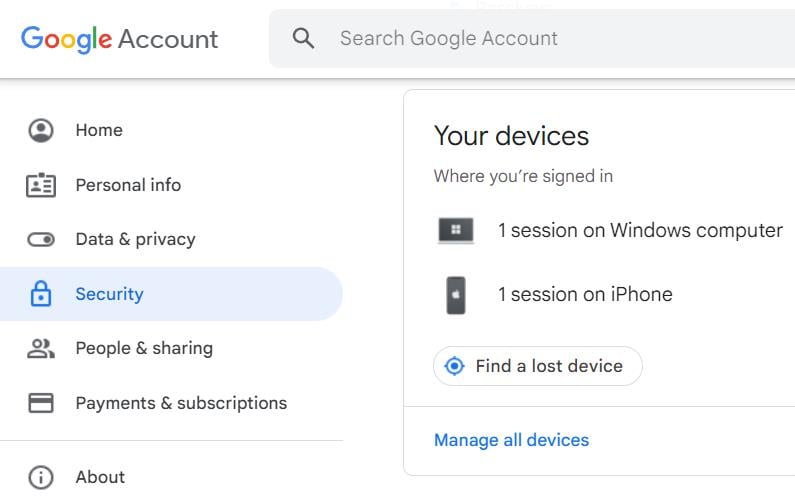A colorful screenshot from a computer display, showcasing the various features available within a Google account. The interface prominently features a search bar at the top, allowing users to quickly locate specific settings or information by typing in key terms. Below the search bar, several navigation tabs are visible: Home, Personal Info, Data & Privacy, Security, People & Sharing, Payments & Subscriptions, and About.

In this screenshot, the user has hovered over the "Security" tab, revealing a detailed list of security options on the right-hand side. These options include: "Your Devices," which shows that there is currently one active session on a Windows computer and another on an iPhone, with links to find a lost device or manage all devices.

The background of the screen is white, with text primarily in black and gray for a clean and straightforward appearance. The iconic Google logo, in its vibrant rainbow colors, adds a splash of color to the otherwise monochromatic interface.